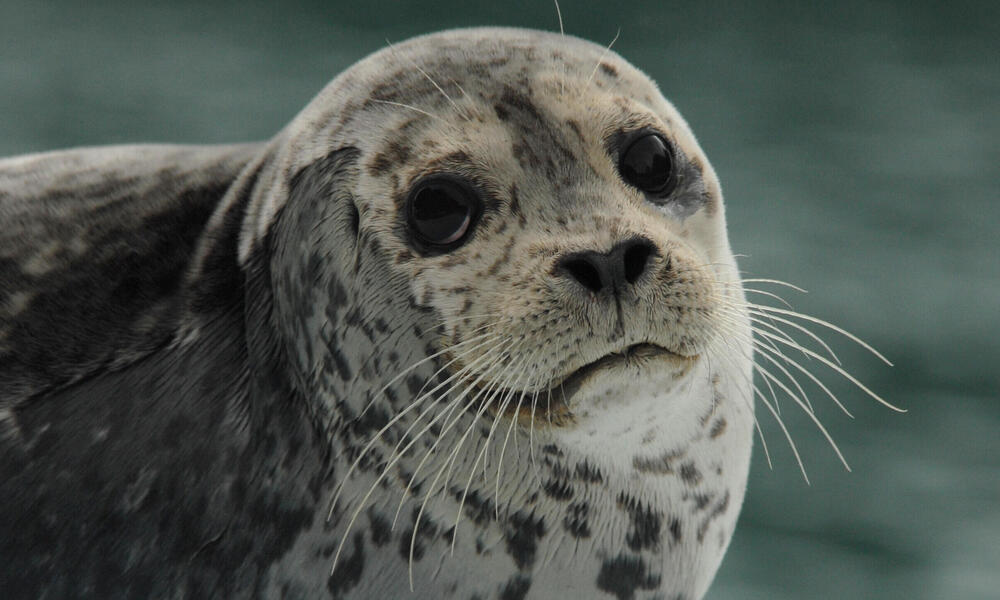In this landscape-oriented color photograph, the subject is a close-up of a spotted seal, centrally positioned with its face taking up most of the foreground. The seal's head, extending down to mid-chest, dominates the frame, while the rest of its body is partially visible and cropped off just below the ribs, extending towards the left. The seal’s fur is a light beige on its face adorned with small brown spots, transitioning to white with the same brown spots on its neck and chest, and dark grey with black spots on its back. Its large, round black eyes, tiny black nose, and white whiskers give it a beguiling, almost pleading expression. The mottled dark greyish-green background is heavily blurred, providing no distinguishable details, effectively focusing attention on the seal's detailed and textured fur. The overall scene appears to be outdoors, capturing the seal in a moment of vivid photographic realism.